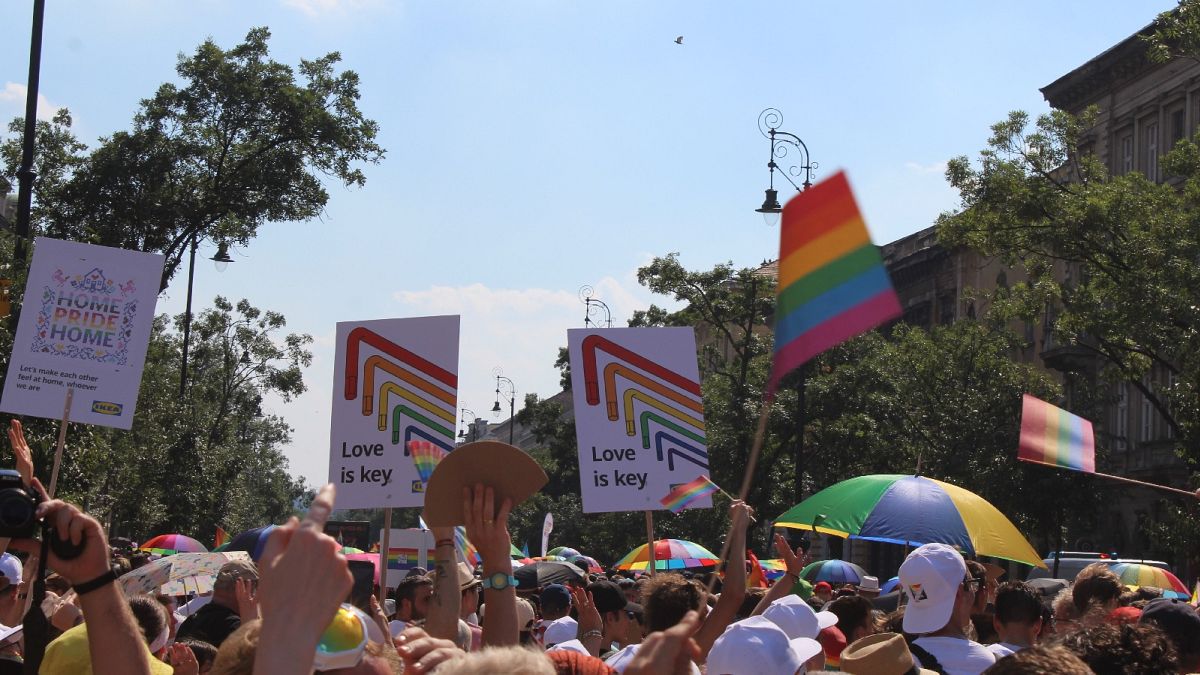This is a vibrant color photograph capturing the energetic atmosphere of a pride parade. The scene is bustling with a large crowd, predominantly showing the tops of people's heads and their colorful banners and flags. The parade participants, who appear to be mostly young adults in their mid-twenties, are holding up pride flags, including rainbow-colored ones, and an assortment of signs. Prominent posters include slogans like “Love is Key” and “Home Pride Home.” There are also unique decorations such as rainbow-colored pipes shaped like sideways L's and rainbow-colored umbrellas adding to the festive ambiance. The backdrop features tall buildings and leafy trees under a sunny sky with barely a cloud in sight, typical of a lively cityscape during a joyful celebration. Similarly, a tall streetlight is visible, further situating the event in an urban setting.